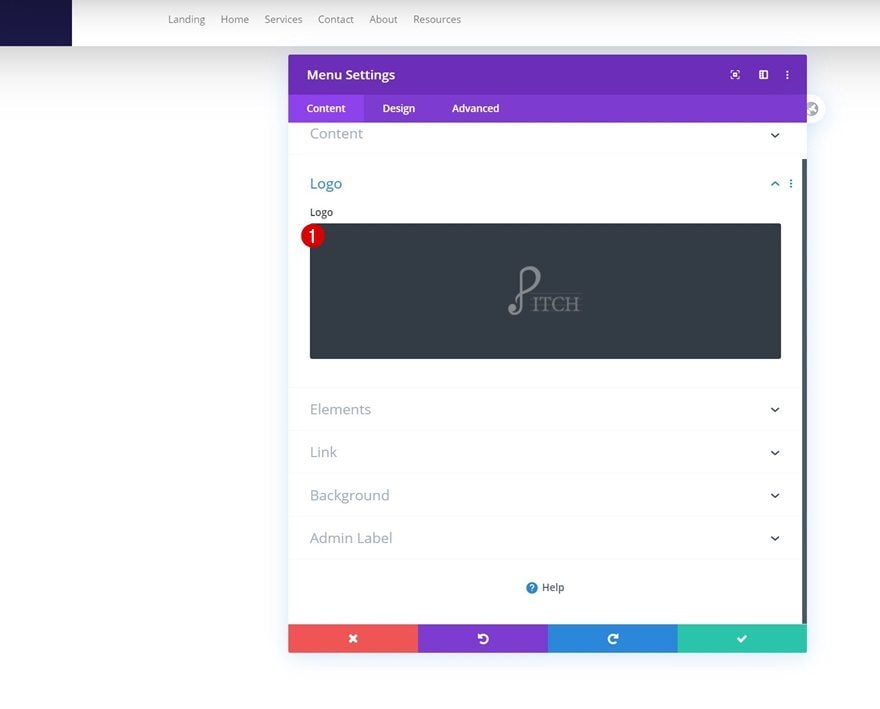This is a detailed digital image capture, possibly taken from a cell phone or computer screen. At the top of the image, there is a navigation bar with a white background and black text. The leftmost text reads "Landing," followed by "Home," "Services," "Contact," "About," and "Resources."

Beneath the navigation bar, there is a purple-tinted box titled "Menu Settings" in white text. The "Menu Settings" section is expanded to reveal several tabs: "Content," "Design," and "Advanced." The "Content" tab is currently selected.

Within the "Content" tab, the first option displayed is "Logo." Underneath this header, the section repeats the word "Logo" in black text. Below, there is a black box featuring a stylized letter 'P' followed by the letters 'I', 'T', 'C', 'H' in uppercase, written in a gray font. A red circle with the number '1' appears next to the word "Logo."

Further down, additional options include "Elements" and "Link," each accompanied by drop-down menus. The menu continues with sections labeled "Background" and "Admin Label." The bottom of the image features a "Help" button. The overall layout and options suggest this is a screenshot of a digital interface, perhaps a website builder or content management system.